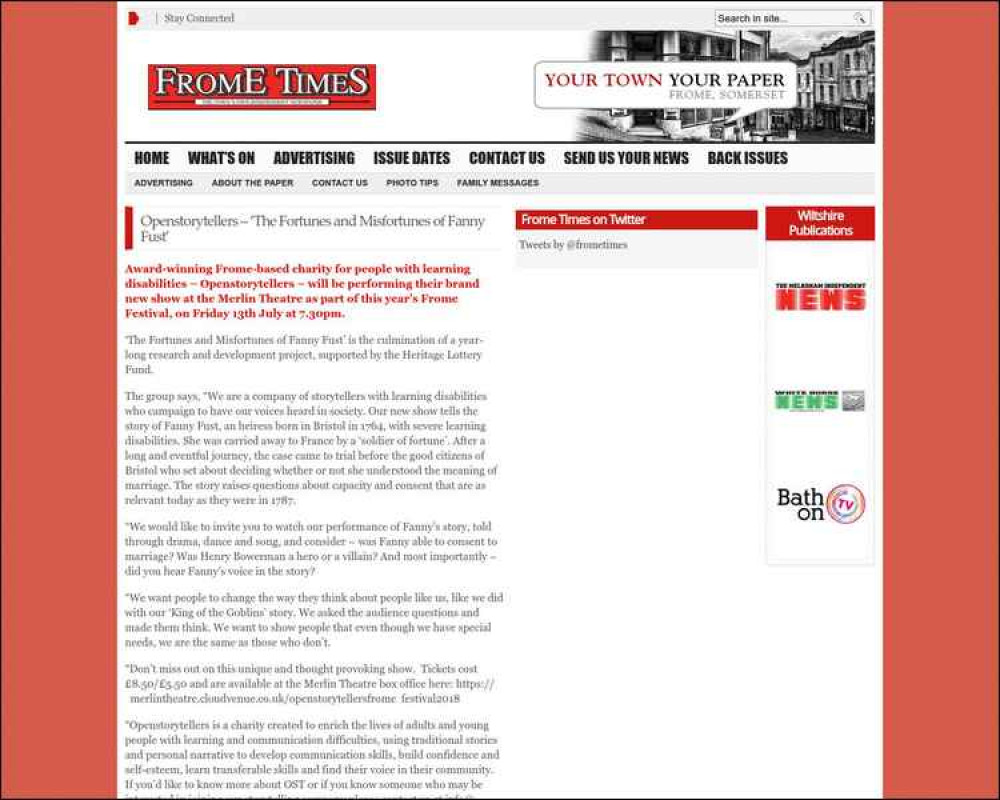**Descriptive Caption:**

The web page features a layout with distinctive bezels in red on both the left and right sides. Dominating the top part of the page is a large white rectangular section. On its left side, there is a gray header with a red mark, accompanied by the text "Stay Connected" in black.

To the far right of this header, another white rectangle includes the bold black text "Search in Sight," and showcases a black-and-white photograph portraying old buildings flanking either side. Atop one of these buildings, a white rectangle with a thought bubble is positioned, containing the red text "Your Town" and bold black text saying "Your Paper." Beneath this, the text "Frome, Somerset" appears in gray font. Additionally, on the left side, the words "Frome Times" are highlighted within a red rectangle.

Below this, a light gray bezel contains a navigation bar with black text reading: "Home," "What's On," "Advertising," "Issue Dates," "Contact Us," "Send Us Your News," and "Back Issues." Multiple clickable buttons underneath this section are labeled as "Advertising About the Paper," "Text Us," "Photo Tips," "Family Messages," all within a dark gray bezel.

Further down, another light gray section features a red line on the left edge, and the black text "Open Storytellers - The Fortunes and Misfortunes of Fannie Fust." There is also red text announcing, "Award-winning Frome-based charity for people with learning disabilities - Open Storytellers - will perform their brand-new show at the Maryland Theater as part of this year's Frome Festival on Friday, 13th July at 7.30 p.m."

To the right of this, "Wiltshire Productions" is mentioned alongside news categories labeled in red and green, and the term "both" appears next to a multicolored TV icon with bands of red, green, blue, and purple. A red rectangle at the top displays white text announcing "Frome Times on Twitter," with black text below that saying "Tweets by @FromeTimes." 

Finally, there is additional black text along the left-hand side of the main body of the page, contributing to the detailed content of the website.